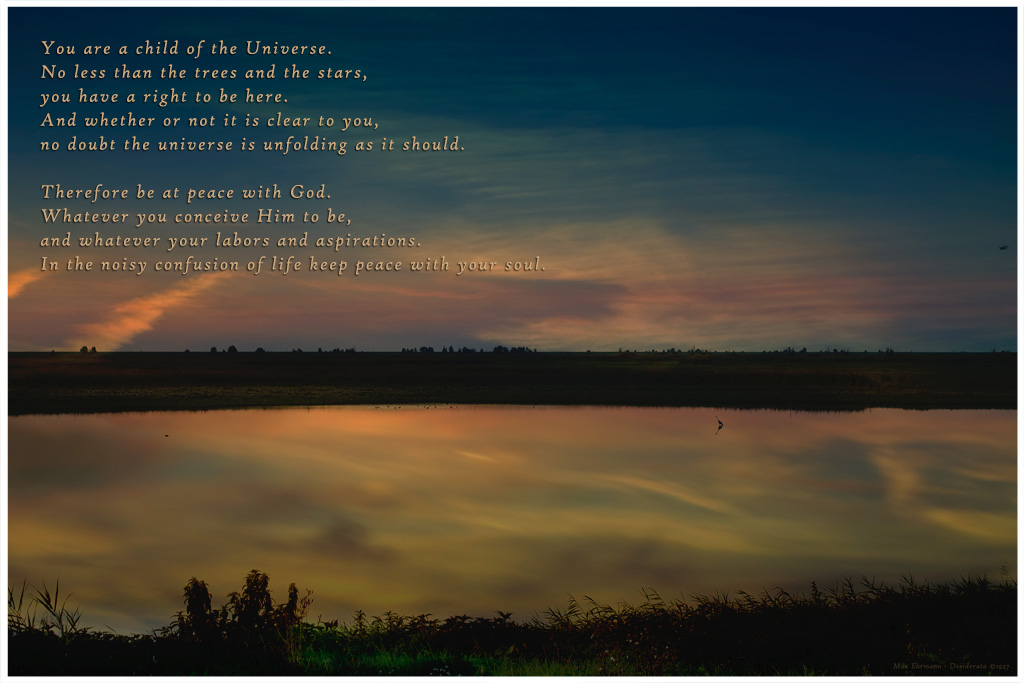The image is a rectangular photograph, akin to something you'd find as a fridge magnet, prominently featured on a webpage, or framed on a wall as a piece of motivational decor. It captures a stunning sunset over a serene, small lake or large pond, surrounded by green grass and bushes. The sky is a vibrant blend of blues, pinks, purples, and oranges, with fluffy white clouds tinged with pink near the horizon, all beautifully reflected in the tranquil water below. A lone grey bird can be seen gracefully floating on the pond. In the top left corner of the image, there is inspirational text, possibly in yellow or white, that reads: "You are a child of the universe, no less than the trees and the stars. You have a right to be here, and whether or not it is clear to you, no doubt the universe is unfolding as it should. Therefore be at peace with God, whatever you conceive him to be, and whatever your labors and aspirations, in the noisy confusion of life, keep peace with your soul."